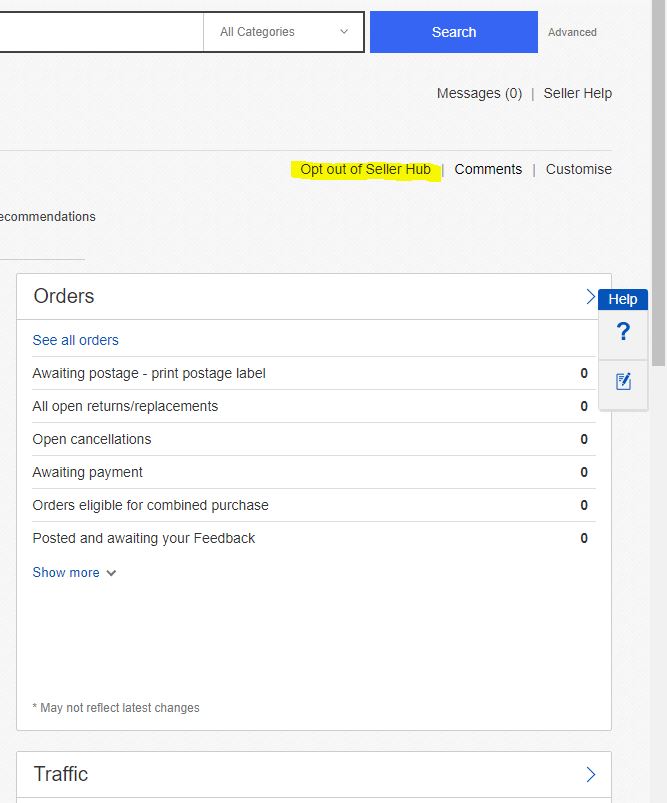The image depicts a segment of a website interface designed for online sellers. The predominant colors are white and gray, with accents of blue. At the top of the page, there are three horizontally-aligned elements. The first is labeled "All Categories" with a downward arrow indicating a drop-down menu. Next to it is a blue rectangle with white text that says "Search." Following that is a section with a gray-white background and the word "Advanced" in gray text.

Beneath the "Search" button is the word "Messages" followed by "(0)," implying that there are no new messages. Next to it, separated by a vertical bar, is the phrase "Seller Help," where the first letters of "Messages," "Seller," and "Help" are capitalized. Below this line, the text "Opt out of Seller Hub" is highlighted. Additional vertical bars separate the options "Comments" and "Customize."

Further down, the website offers more navigational options, likely related to managing the backend functionalities for sellers. Tabs like "Orders" suggest areas where the user can manage different aspects of their online sales.